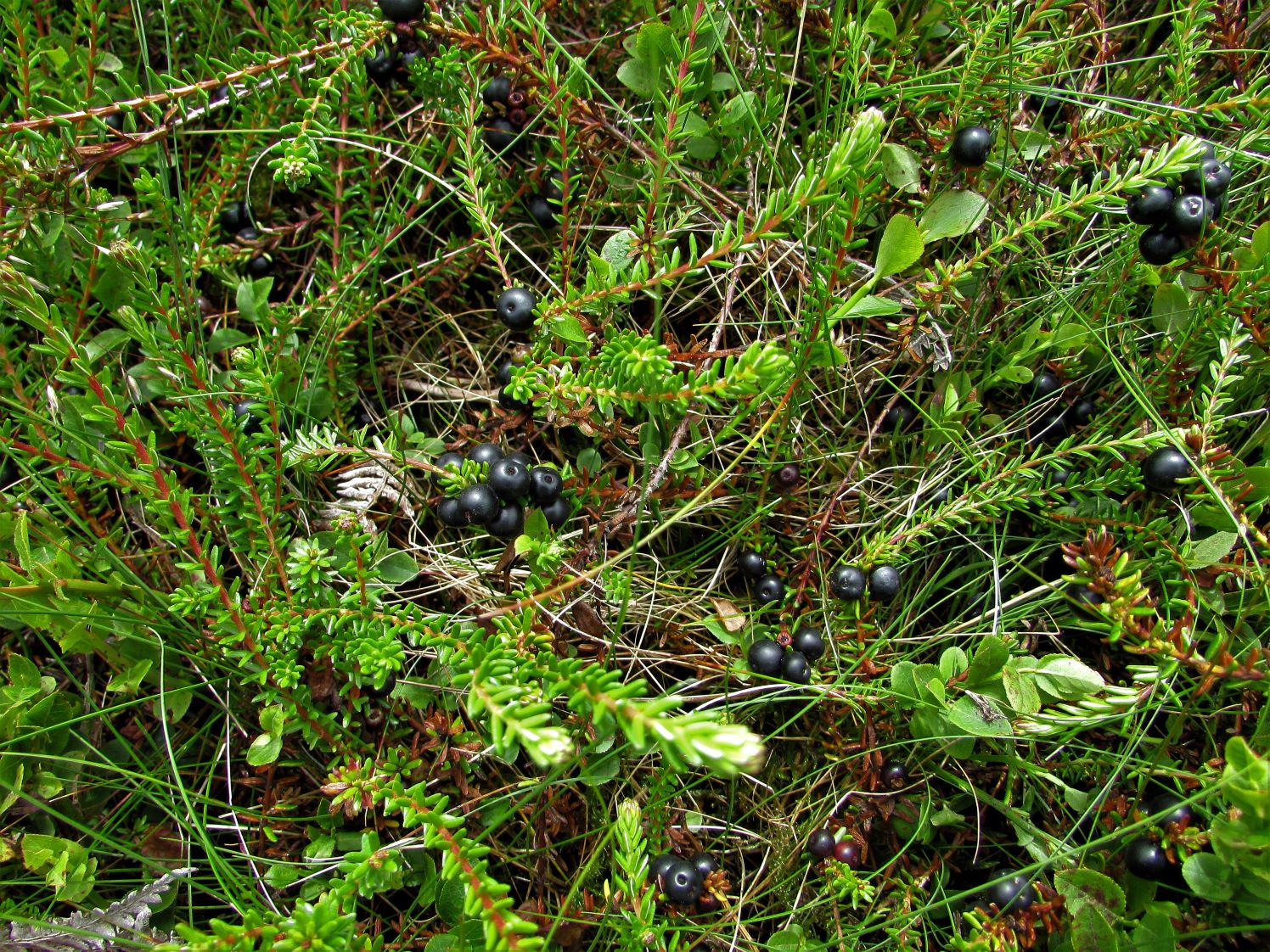This close-up image captures a seemingly wild blueberry bush. The dense greenery overwhelms the scene with its bright, lively hue, interspersed with intertwined brown stems and occasional patches of dry grass. The tangles of green limbs, small leaves, and old, dead sticks give the impression of late season growth. Shiny, plump, and very dark blueberries border on black and are notably scattered, concentrating mainly in the center and top-right areas of the image. Although the sun itself isn't visible, its presence is implied by the sunlit green leaves, suggesting a sunny day. The bush's intricate and messy appearance makes it unclear if the plant is grounded or part of a larger thicket.